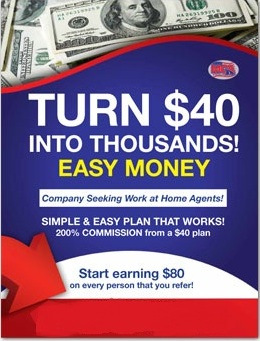The image features an old-school advertisement that seems to promote a money-making scheme targeted at work-at-home agents. Dominating the blue background is large white text proclaiming, "Turn $40 into Thousands! Easy Money." The phrase "Easy Money" stands out in bright yellow font, adding emphasis. Below this, the ad elaborates on a simple and easy plan that works, with a promise of a 200% commission from a $40 plan, and highlights, "Start earning $80 on every person that you refer." This phrase is underscored by a red arrow pointing towards it and is set within a white section framed by a red border. Surrounding the text, the ad features clipart images of $100 bills, giving the impression of piles of cash, reinforcing the get-rich-quick promise.